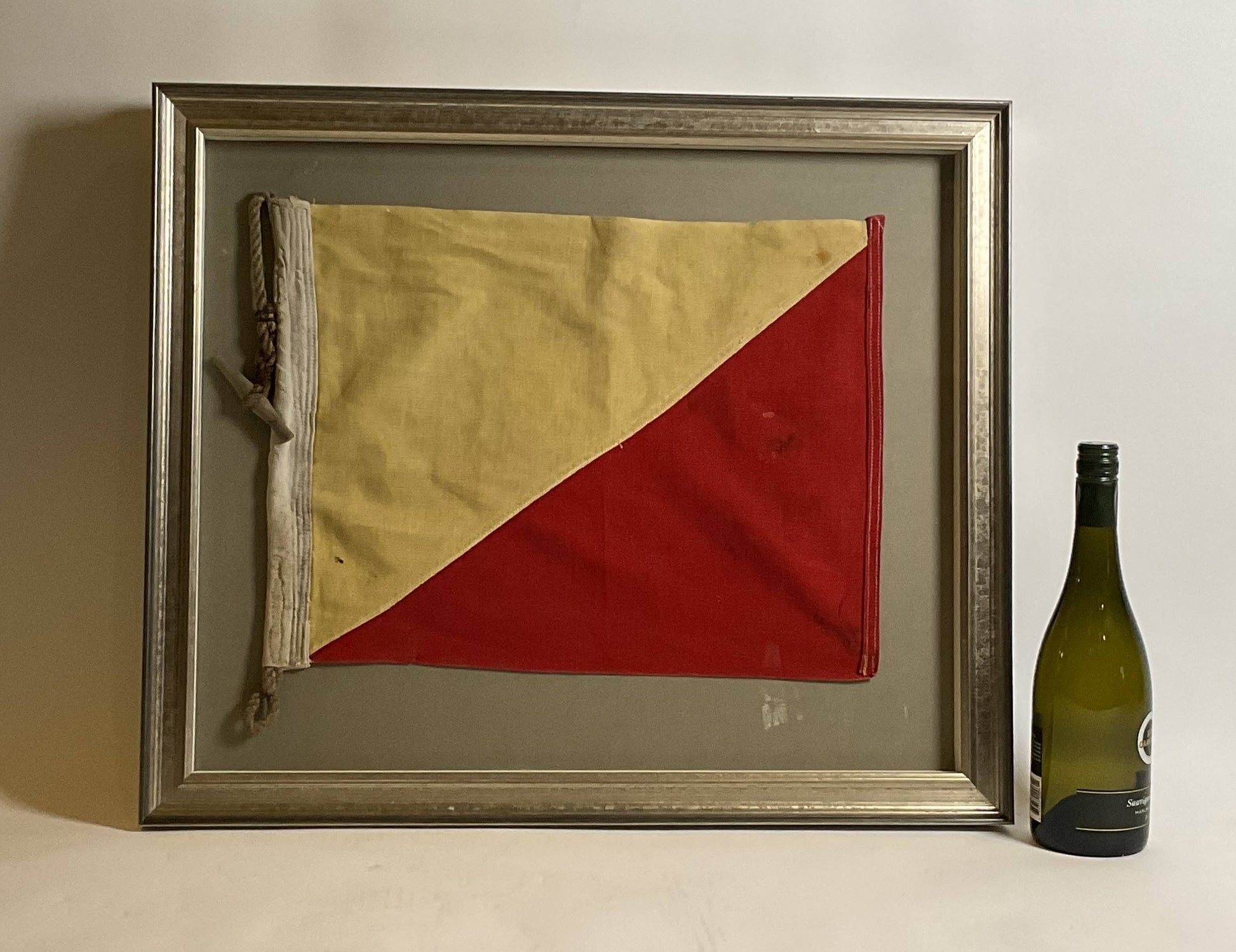In the photograph, a vintage, discolored flag is showcased within a slightly battered gilded frame, all set against a plain off-white background. The flag is divided diagonally from the top right to the bottom left, creating two triangular sections, with the top left being yellow and the bottom right being red. The frame contains additional details like a piece of white cloth, tied through with a rope that hangs alongside it, and a small piece of wood at the end of the rope. To the right of this framed flag, an empty green wine bottle with a black stopper stands. The bottle’s label is partially obscured and rendered unreadable, but features black and white colors. The overall scene appears to be captured in a museum-like setting, where the objects are centrally positioned with a focus on the framed flag, and a light source illuminates through the clear green bottle, emphasizing its contents and color.